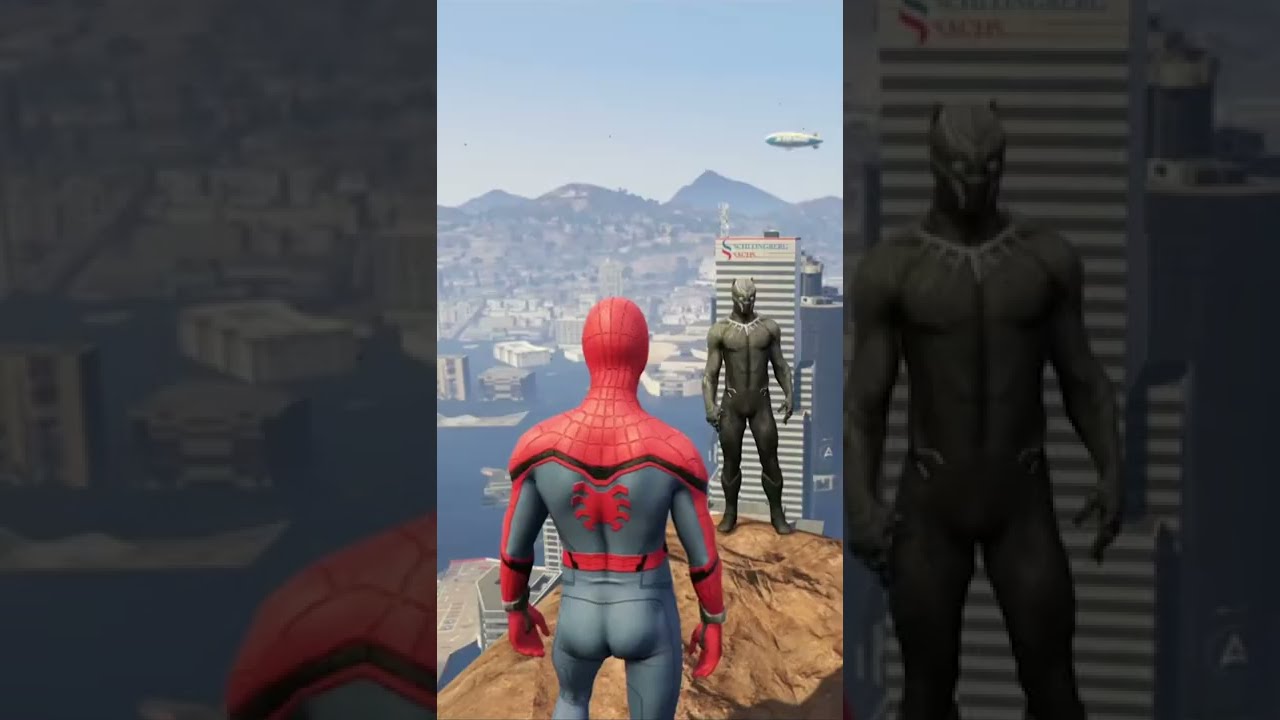The image is a detailed graphic composed of three vertical portrait panels arranged in a landscape orientation. The center panel showcases the primary scene: Spider-Man, depicted from the hamstrings up in a red mask and blue suit with red spider insignia, red belt, red sleeves, and red gloves, standing on a rocky outcrop. He's facing off against a villain donning a black suit, a spiked necklace resembling stalagmites, and a mask, reminiscent of the Black Panther's attire. The left and right panels are close-up details of the central image, overlaid with a black opaque background to fit the landscape format.

Spider-Man and his adversary are perched high above a city, with skyscrapers and water visible below, and a mountainous landscape in the backdrop. The sky is blue, featuring a floating blimp, adding to the dramatic atmosphere. The graphic, which could be from a video game or a detailed digital artwork, conveys the high-stakes tension of a standoff between hero and villain on a precipice above the urban sprawl.